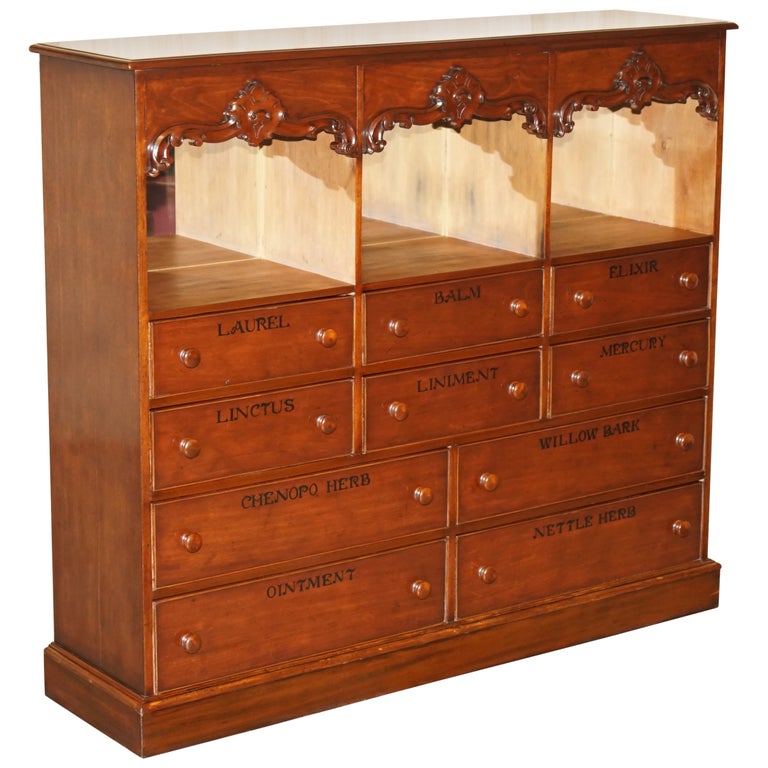The image depicts a vintage apothecary's chest made of dark wood, accentuated by honey-colored panels near the top, giving it a classic and rustic vibe. The upper section of the chest features three open cubby holes adorned with a decorative border. Below these are multiple rows of drawers: two rows of three drawers each, followed by two rows of two drawers each. All the drawers have round handles for easy pulling. Labeled in black across the fronts of the drawers, you can read terms associated with old-fashioned remedies, such as "laurel," "balm," "elixir," "lenctus," "liniment," "mercury," "chinopo herb," "willow bark," "horn ointment," and "nettle herb." The labels suggest that the chest was used for storing various herbs and concoctions typical of early medicinal practices.